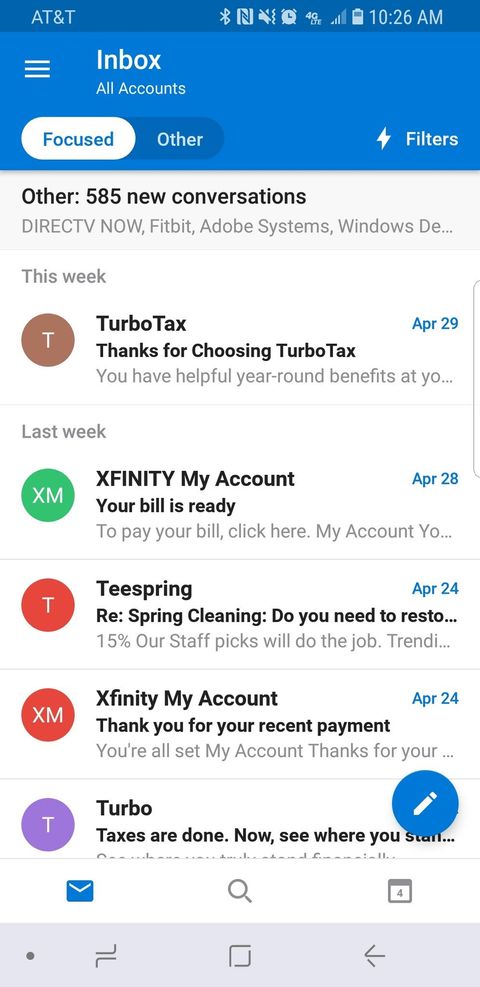This image displays a user's smartphone screen featuring a landing page for an email application. At the very top, a thin navy blue banner is visible, displaying "AT&T" in white text on the left. The right side of this banner shows various status icons, including a battery icon indicating roughly 50% charge and the current time: 10:26 AM.

Below this, a wider bright blue banner features the text "Inbox, All Accounts" in white. Directly underneath, two buttons allow the user to switch between "Focused" and "Other" inbox views, with "Focused" currently selected. To the right of these buttons is the word "Filters" also in white text.

Following this, a light gray ribbon appears, displaying "Other: 585 New Conversations" in black text. Below this ribbon, there are several entries listed in gray text: "Direct TV Now," "Fitbit," "Adobe System," and "Windows." On a white background under these items, "This Week" is written in light gray text.

Below "This Week," an email from TurboTax is prominently displayed. "TurboTax" appears in black text, followed by "Thanks for choosing TurboTax" in black, and the beginning of the email preview in light gray: "You have helpful year-round benefits at your." The email date, April 29th, is shown in bright blue.

Further down the screen, a section labeled "Last Week" appears, followed by a list of emails.